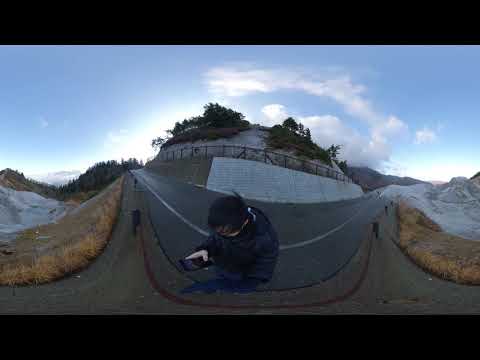The image presents a vertical, rectangular scene viewed through a door's peephole, giving a warped, bent perspective. In the center stands a person with dark hair, clad in a black jacket and dark blue jeans, their head bowed as they focus on a black cell phone held in their right hand. The street they're on curves like an upside-down U or rainbow, with a white stripe dividing the dark pavement. Behind the person, a fence rests atop a retaining wall, enclosing a hillside with gray stone and rocky outcroppings. The hillside has green shrubs and some scattered trees at the top, adding to its rugged look. On the left and right sides of the image, the landscape features grassy inclines and more rocky and gray dirt areas, leading up to further hills adorned with trees. The sky above is a clear blue with a few white clouds, and the entire scene is framed by a thick black border at the top and bottom.